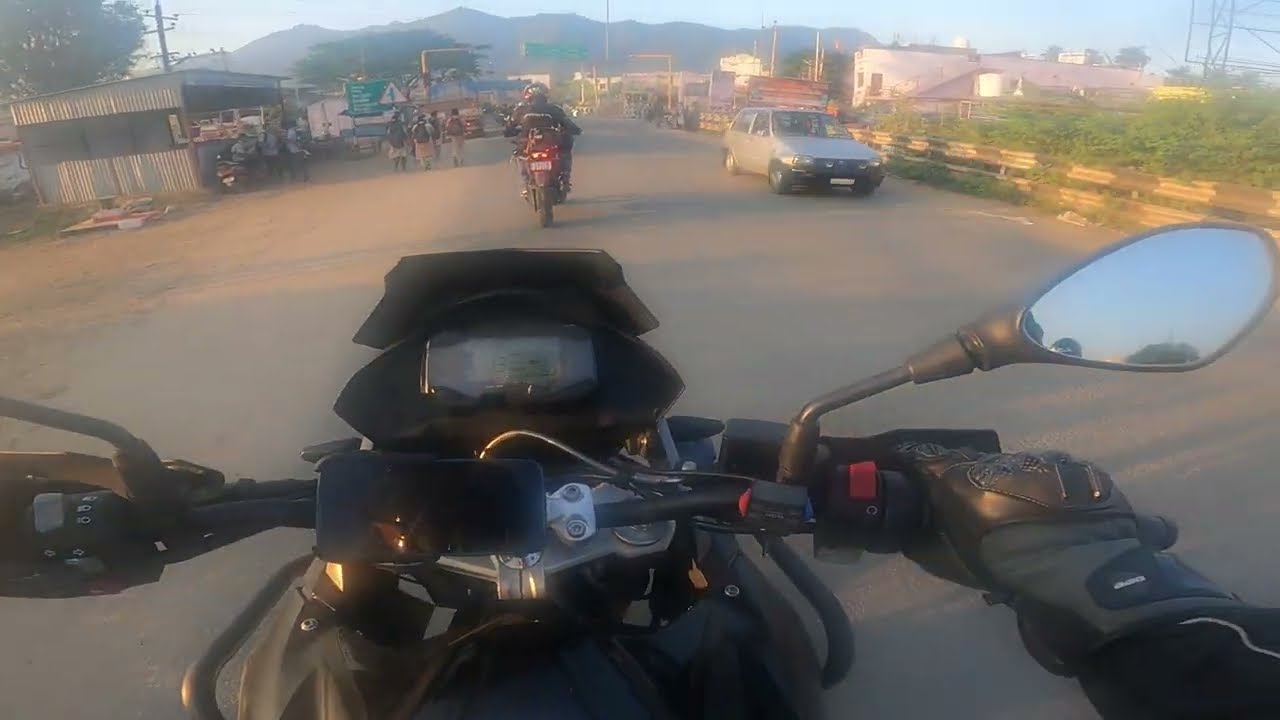This image captures the view from a motorcyclist's perspective, riding along a wide, unmarked asphalt road that eventually transitions into a dirt path. The foreground of the photo is dominated by the black dashboard of the motorcycle, showcasing an array of wires, gadgets, and a smartphone mounted on a metal arm. A black-gloved hand grips the handlebars, extending from a sleeve of a matching black jacket. On the right side of the motorcycle, a side view mirror reflects a clear blue sky.

Ahead, another motorcyclist in a black jacket and helmet leads the way, their taillights glowing red, indicating they are braking. To the right, a small silver four-door hatchback car approaches, with greenery and a fence separating the road from a long pink sandstone building behind it. Further right, there's a large white structure flanked by green bushes.

On the left side of the road, a group of kids with backpacks and several people walk alongside a corrugated tin structure, which resembles a bus stand. Behind them, additional shanty-like buildings can be seen. The horizon is adorned with thickly forested mountains, under an expansive blue sky. The photograph is somewhat gray and faint, adding a nostalgic or gritty quality to this scenic, outdoor daytime setting.